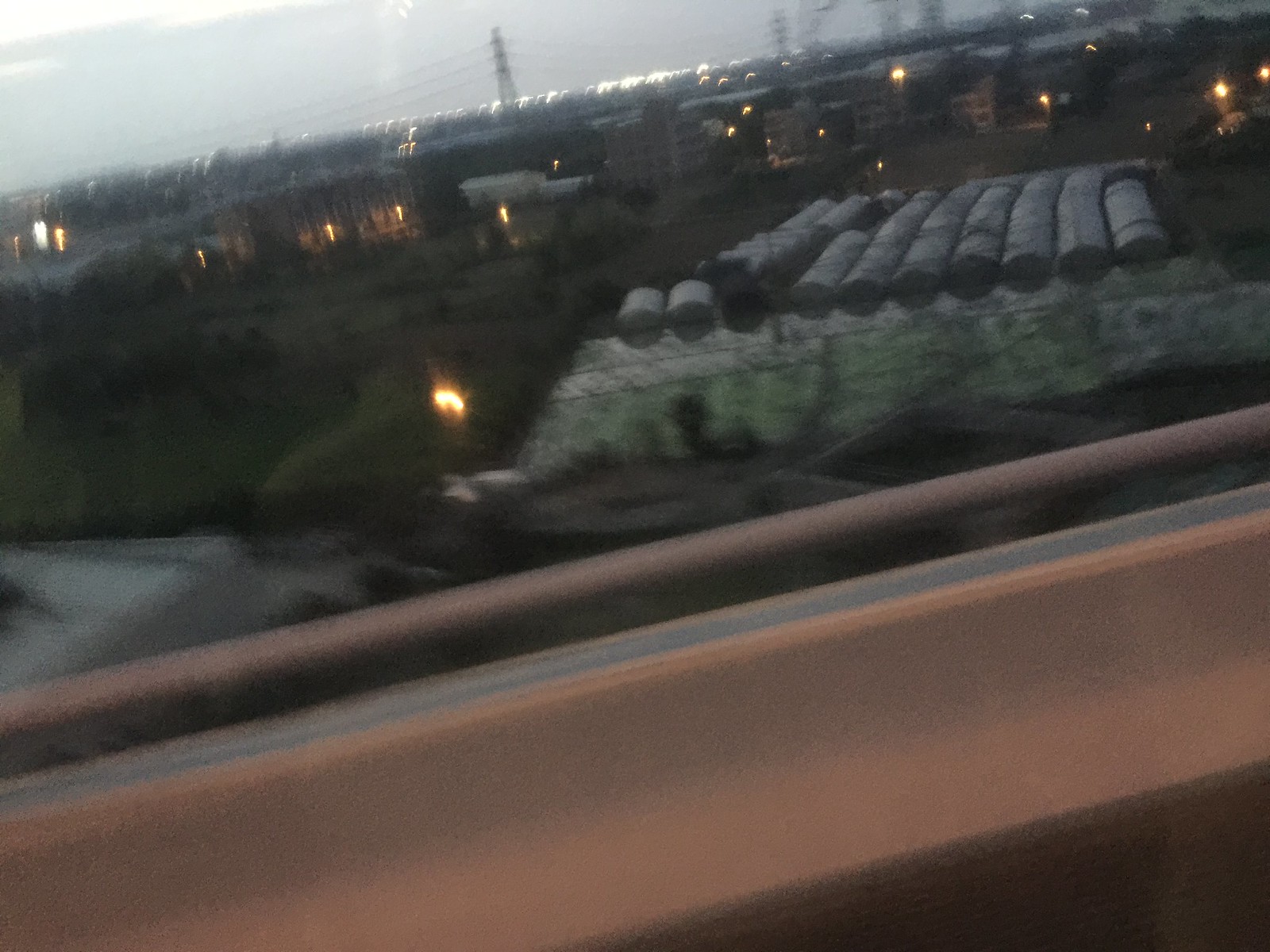This color photograph, taken outdoors just before dark, captures a blurred image likely shot from a moving train or other form of transportation. In the foreground, a white rail stretches across the bottom. The scene behind it is a sprawling industrial complex with various elements visible. The railroad track running through the image appears slightly rusted. To the right, a train yard houses multiple trains, automobiles, and orderly stacked silver steel drums. Tall electrical power towers with heavy, sagging lines connect across the yard, contributing to the industrial environment.

The landscape is dotted with multi-story buildings, dirt patches, and bushes, all illuminated by orange lights as evening approaches. The sky remains clear but darkens progressively, with city lights twinkling faintly in the far background. A fence encloses parts of the yard, adding to the industrial aesthetics. Grass areas and other miscellaneous items are scattered throughout, enhancing the richness and detail of the bustling scene.